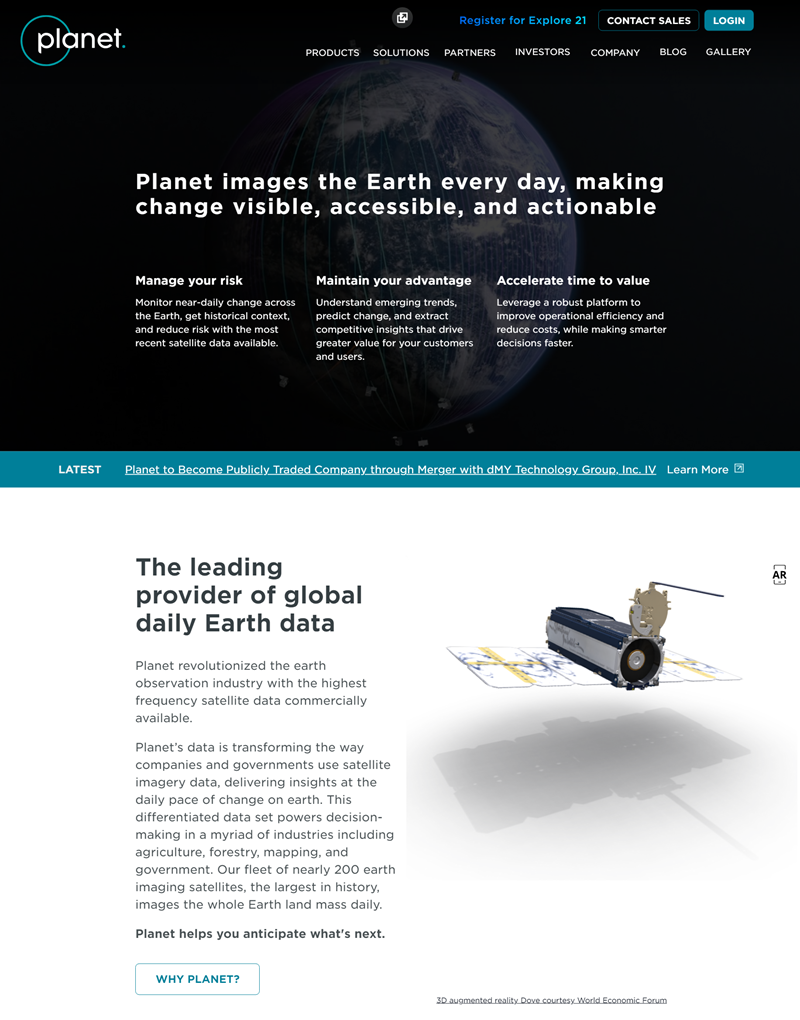**Descriptive Caption:**

The image displays an online webpage designed to resemble a rectangular portrait, divided into two primary sections.

**Top Half:**
- **Background**: The upper section of the webpage features a predominantly black background with a bluish-teal footer strip at the bottom.
- **Logo and Header**: In the upper left, the word "planet" appears in lowercase white text with a teal circle logo situated behind the “A” in "planet".
- **Slogan**: Centered in white text, the slogan reads across two lines: "planet images the earth everyday, making change visible, accessible, and actionable."
- **Subsections**: Below the slogan, three subsection headers in bold white read: 
  - "Manage Your Risk" 
  - "Maintain Your Advantage" 
  - "Accelerate Time to Value"
  Each subsection has four to five lines of detailed, left-justified white text.
- **Navigation and Buttons**: To the right of the logo are two rows of headers:
  - **Top Row**: 
    - "Register for Explore 21" (medium blue)
    - "Contact Sales" (thin black box outlined in white)
    - "Login" (teal rectangular box with rounded corners).
  - **Second Row**: Seven clickable headers labeled: "Products", "Solutions", "Partners", "Investors", "Company", "Blog", and "Gallery" (all caps, white font).
- **Footer Section**: The bluish-teal footer has white text. In the lower left:
  - Bold text reads, "LATEST IN".
  - Underlined text next to it states, "Planet to become publicly traded company through merger with DMY Technology Group Inc. IV."
  - Adjacent to it, the phrase "Learn more", not underlined.

**Bottom Half:**
- **Background**: This section has a white background with no borders.
- **Text**: Toward the left, indented, a three-line header states, "The Leading Provider of Global Daily Earth Data".
  - Two paragraphs follow; the first is about three and a half lines, the second approximately eleven lines.
  - At the bottom, a bold sentence reads, "Planet helps you anticipate what's next."
  - Below this, a clickable teal outlined box with teal text says, "WHY PLANET?"
- **Image**: To the right, there is a portrait rectangular image of a floating digital object resembling a camera, likely representing a satellite. It appears silver and black, tubular with bars on top, casting a shadow beneath on a rectangle resembling computer chips.

This detailed layout effectively showcases Planet’s online presence, highlighting their services, brand identity, and navigational elements.